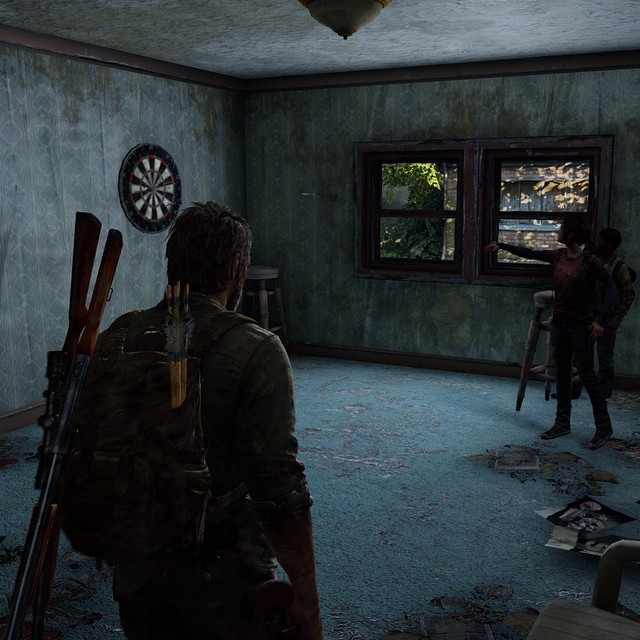In this animated still image from "The Last of Us," the scene unfolds in a dimly lit, dilapidated room that resembles a neglected basement. The walls are gray and dirty, with peeling paint and shadowy discoloration. A dartboard is mounted on the far wall, near two children—Ellie, a young white girl in a red shirt and dark pants, and Sam, a smaller African-American boy. Ellie is in the motion of throwing a dart, which is visibly airborne. Both kids have backpacks with visible straps. 

Standing closer to the viewer, a bearded man with short, salt-and-pepper hair watches the children. He has a rugged appearance, wearing dark clothing, a jacket, and a military-like backpack. Strapped to his back are two guns and a set of arrows. His right sleeve is rolled up, emphasizing his readiness. The room is cluttered with various debris and papers scattered on the worn-out floor. 

Illuminated by daylight filtering through two windows, a glimpse of another house and some greenery are visible outside. Despite the presence of a ceiling light, it remains off, adding to the room's rustic, uncared-for ambiance. The sparse furnishings include a couple of stools, adding to the sense of abandonment and disuse in this hauntingly detailed game environment.